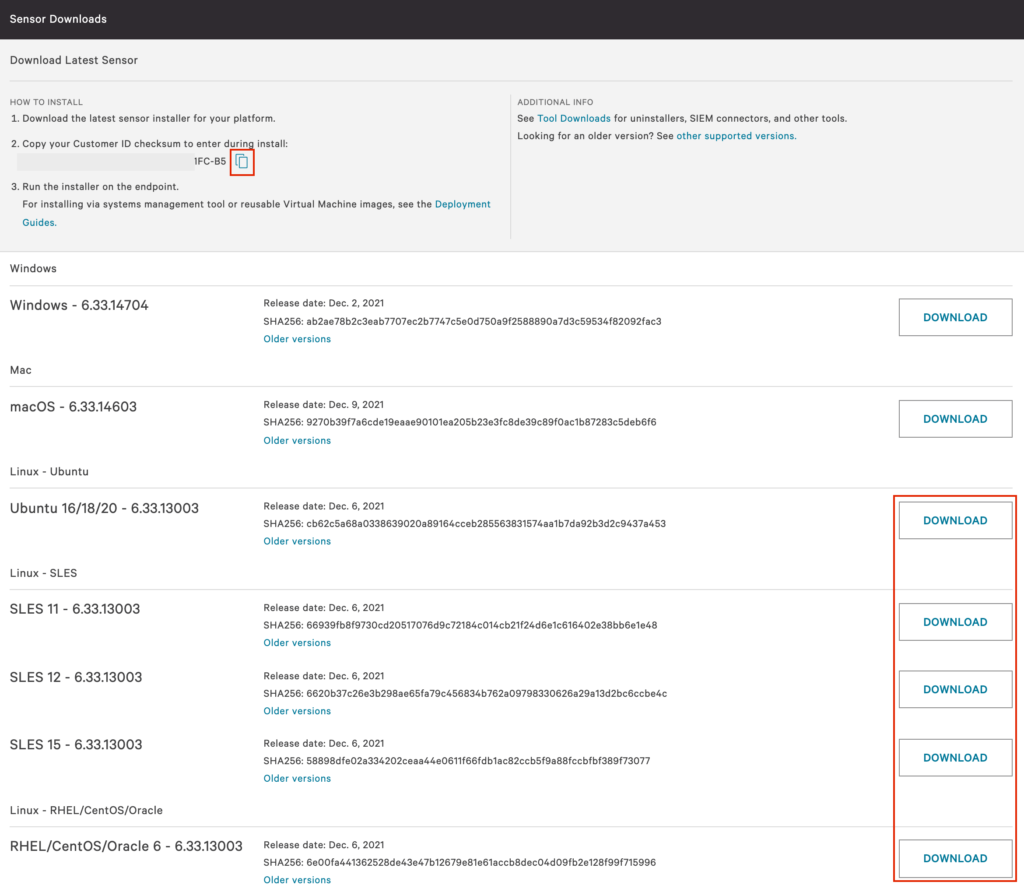The image features a primarily white background. At the top, there's a black box labeled 'Sensor Downloads.' Below it, two blue boxes are displayed: the first one, smaller in size, is labeled 'Download Related Sensor,' while the second box provides instructions on 'How to Download and Install the Sensor.'

Adjacent to these, a red box contains several smaller blue boxes within it. There is also a blue section labeled 'Guides,' and a smaller blue box on the left titled 'Additional Info,' which contains text in blue. 

Further down, a section indicates the words 'Windows' with a dividing line beneath, followed by the version information 'Windows 6.33.14704'. Alongside this information is a blue 'Download' button.

Additional OS-related sections are marked with 'Mac OS' and 'Linux,' each followed by the version details in blue text. For instance, 'Ubuntu 6.18.20' is listed under the 'Linux' section with the corresponding 'Download' button next to it. The 'SLES' Linux versions—SLES 11, SLES 12, SLES 15—also have download buttons, each enclosed within a red square for emphasis. 

At the bottom of the image, further Linux distributions are listed, including 'Linux RHEL', 'Cosmos Oracle', and 'RHEL / CentOS Oracle 6,' each accompanied by a red-highlighted download button. 

Overall, the image presents a structured layout of various operating system versions and detailed download options within a neatly organized interface.